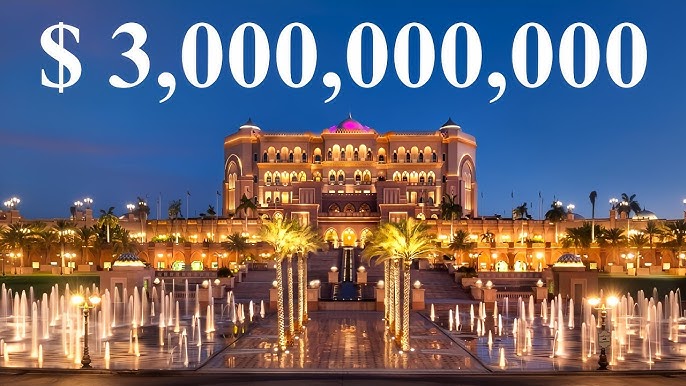The image features a grand, opulent palace that exudes a Turkish or Arabic architectural style, reminiscent of the Taj Mahal. This majestic building, bathed in golden light, stands against a deep blue sky transitioning to dusk, suggesting the remnants of a sunset on the horizon. The palace structure is adorned with numerous oval windows illuminated from within, and it features a prominent pink dome at its center. Below this, the building's massive base ascends from a wide, wet brick pathway lined by rows of palm trees, four on each side. These trees, highlighted by golden lighting, lead to staircase steps that add to the grandeur of the scene. On either side of the pathway, multiple fountains shoot water into the air, reminiscent of the Bellagio fountains. Dominating the top of the photograph in large white letters is the inscription "$3,000,000,000," suggesting the staggering cost associated with this luxurious edifice.